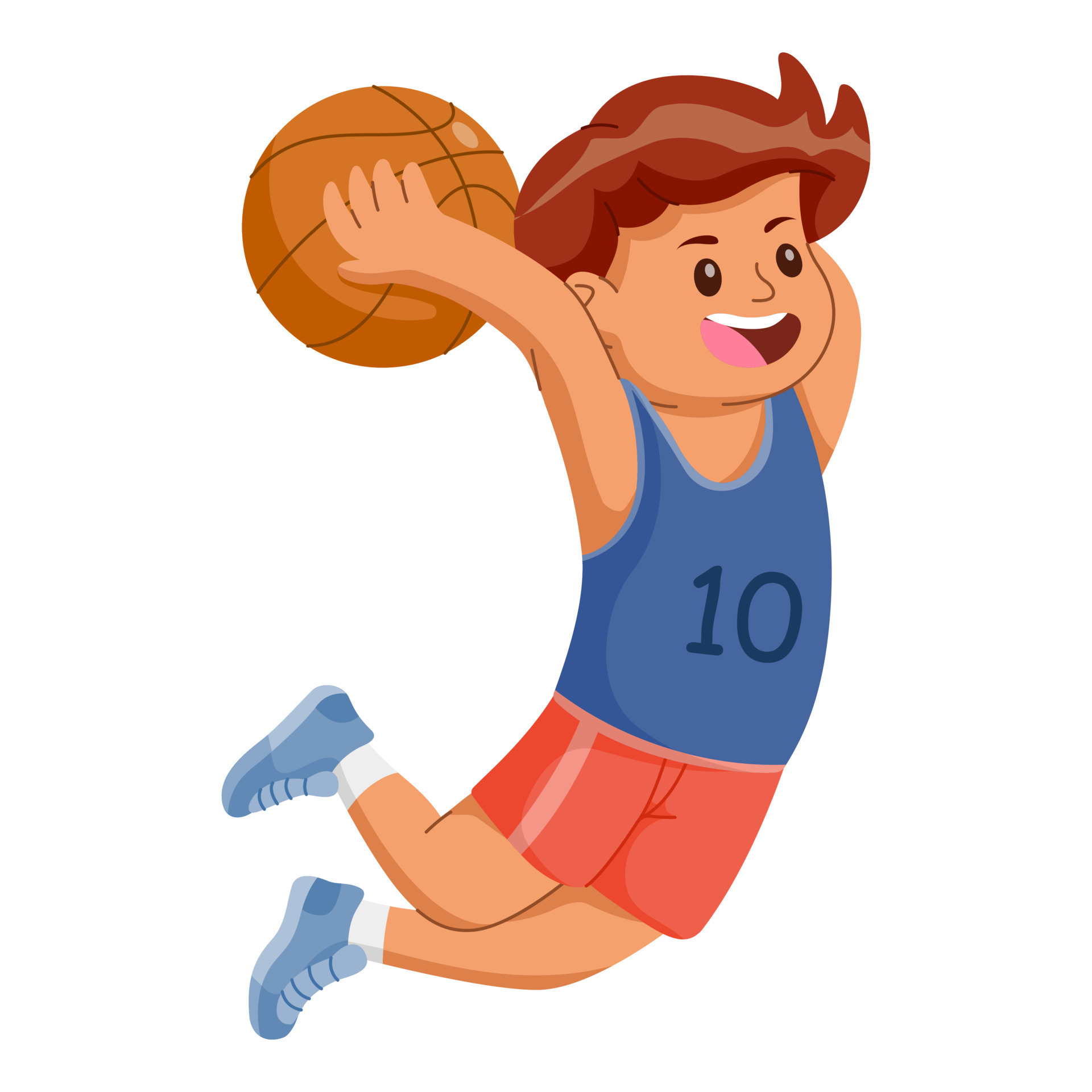This is a detailed digital artwork of a young cartoon boy playing basketball. The boy is depicted in mid-air, seemingly executing a jump shot with an orange basketball in his raised hands. He has medium-length, wavy brown hair, with two wavy portions at the front resembling shark fins. His light brown skin contrasts with his expressive face, featuring black eyes, brown eyebrows, an open mouth showing his white teeth, and a pink tongue. He is donned in a blue sleeveless basketball jersey with light blue lining and the number 10 prominently displayed in darker blue on his chest. Complementing his attire, he wears red shorts with a pink stripe down the sides. His footwear includes stylish blue-colored trainers paired with white socks. The boy's dynamism is emphasized by the white background, which makes the vivid colors of his attire—blue, red, shades of brown, and accents of black and white—stand out even more.